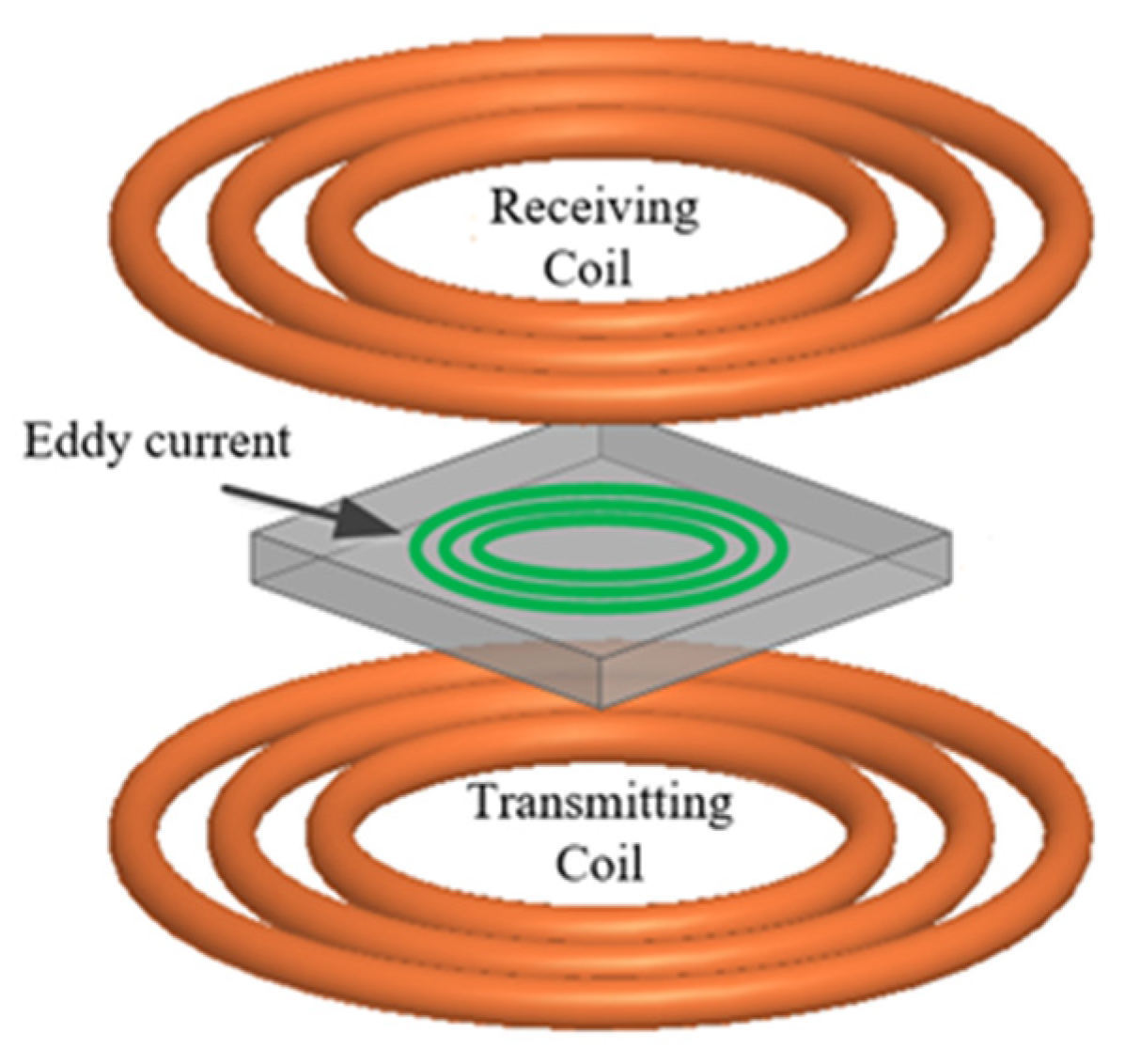This image is a detailed diagram illustrating electrical components, specifically coils and currents. At the top of the diagram, there's a prominent yellow circle stretching across the top third of the image. Inside this yellow circle, positioned slightly down and angled, is a series of three overlapping orange coils identified by the black text "receiving coil" written in the center of a white space within. Below this, a gray tray-like structure houses three concentric green circles, labeled "eddy current" with an arrow pointing directly at these circles. The green circles start larger from the outside and get smaller towards the center. At the bottom of the diagram, similar to the top setup, there's another set of three overlapping orange coils labeled "transmitting coil" in black text within a white center. The colors used in the diagram are primarily orange, green, and gray, with all text labeled in black, providing a clear visual distinction between the receiving and transmitting components as well as the eddy current dynamics in the central gray tray.